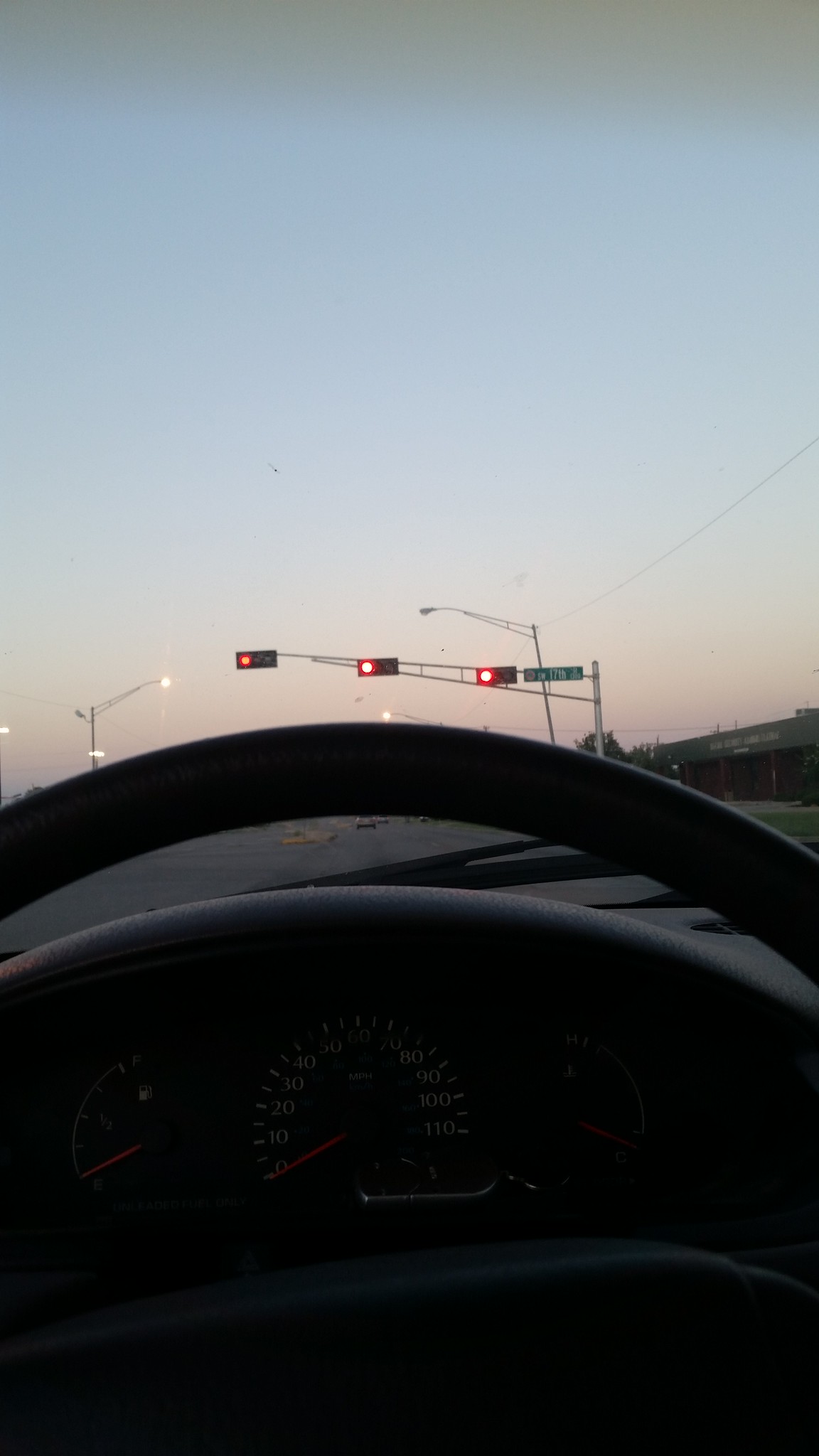This photo, taken from the driver's side inside a car, showcases a detailed view of the vehicle's interior and the exterior surroundings. Inside, part of the steering wheel and the dashboard are visible, featuring the RPM gauge, speedometer (showing zero miles per hour), and gas gauge, all slightly shadowed. Outside, the sky is in a hazy gradient of blue turning to pink, indicating either sunset or sunrise. Prominently, three red traffic lights hang from a metal pole connected to a green street sign that reads "17th Street." Two light poles can be seen in the distance; one is brightly lit while the other remains dark. Power lines run through these lamp posts. On the right side of the photo, there's a short wall along the sidewalk and a building with a green roof.